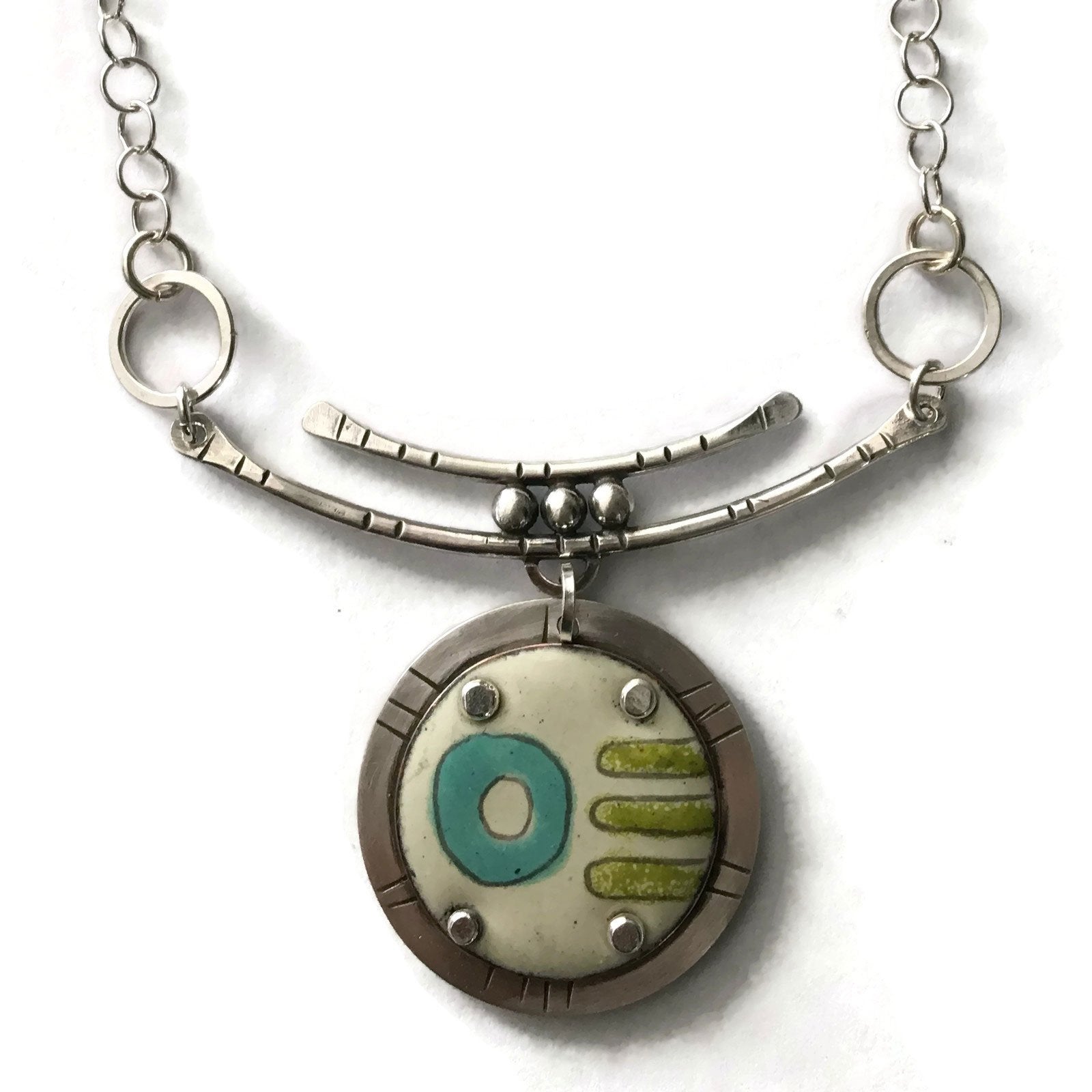The image depicts a striking necklace with a tribal-inspired design. The necklace features a silver chain with several interlinked circular segments, which connect to an arc-shaped silver component. This arc component supports three stainless steel balls and is crowned by a smaller, elevated arc. Suspended centrally from this assembly is a distinctive medallion. The medallion has a circular, possibly bronze or copper-colored frame etched with clusters of lines in various groupings. The interior of the medallion showcases a white inlay that houses a prominent turquoise circle and three horizontal lime green oval shapes. Additionally, there are four silver rivets embedded within this area, adding to the intricate detailing. The pendant's overall color scheme is primarily silver, accented with the vibrant pops of turquoise and lime green, making it a captivating accessory.